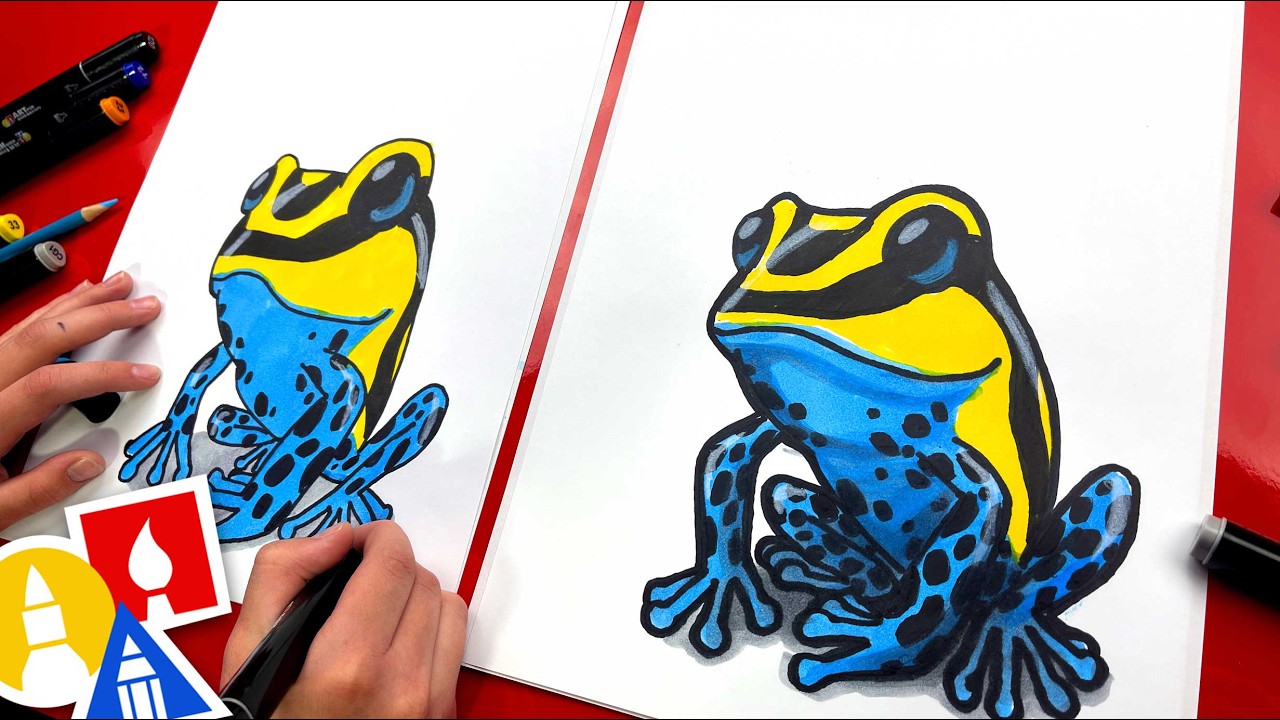This detailed photograph captures the creative process of an artist, likely a teenager, diligently drawing a colorful frog, using a range of vivid colors such as yellow, blue, and black. The image is in landscape orientation and depicts two nearly identical frog illustrations side by side. The frog on the left is less complete, while the one on the right showcases more refined shading and highlights. The artist’s hands are prominently featured near the bottom left corner; the left hand holds the paper steady on a red table, while the right hand wields a black marker. These youthful hands, whose age might suggest a teenager or potentially an adult with young-looking hands, focus intently on their work. The intricate illustration includes detailed elements like a blue belly, black spots, and yellow stripes on the frog. The bottom left corner also features three distinct logos: a gold circle with a white bell tower, a red square with a white candle flame, and a blue triangle with a white pencil point. Scattered colored markers are visible on the top left, hinting at the tools used for the artwork. The overall scene is set against a vibrant red backdrop.